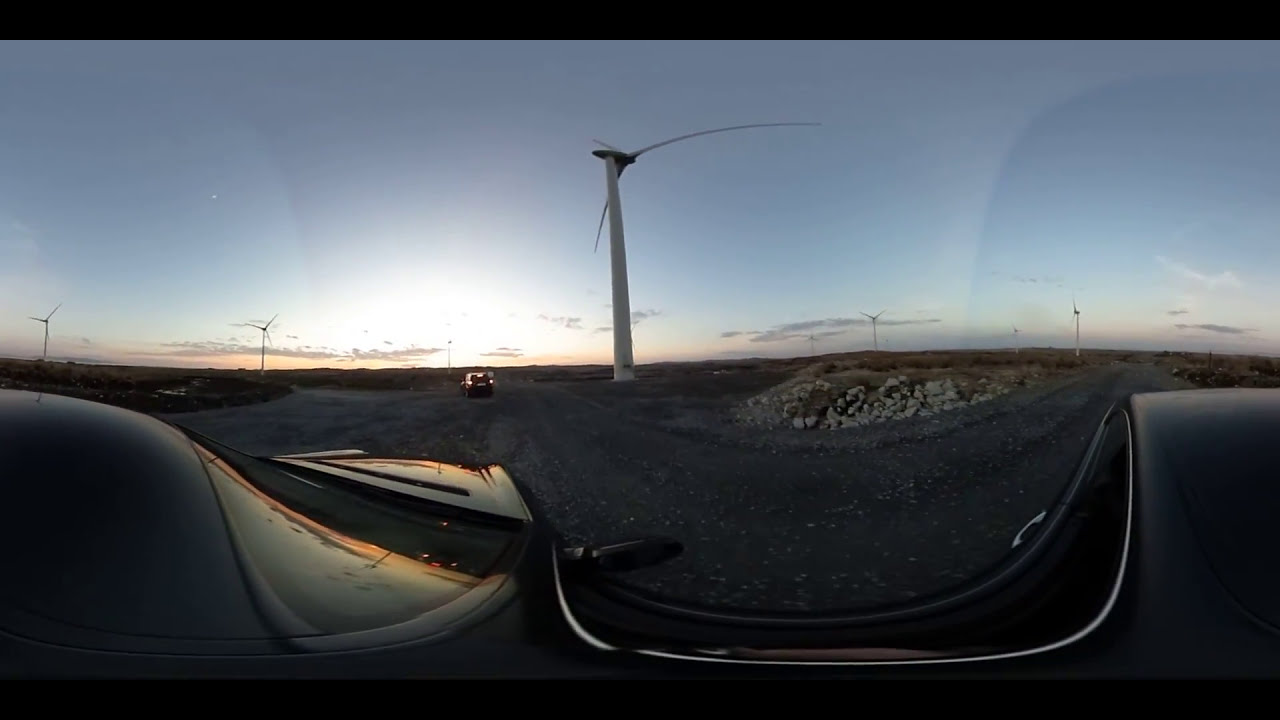The photograph captures a striking scene of a modern white power-generating windmill with three blades, standing prominently in the center and shooting up into the sky as the sun begins to set, casting a warm orange, yellow, and blue hue. The panoramic perspective, likely taken from a moving car on a gravel road, adds a dynamic sense to the composition, creating slight distortion. To the right, rocks are visible, while to the left, some autumnal greenery can be spotted. The unpaved road also hosts another vehicle ahead, partially visible with shiny black surfaces reflecting the evening light, hinting at the presence of another photographer. In the distance, a line of four additional windmills gradually diminishes in size, illustrating depth and emphasizing the expansive landscape. The sky, adorned with few clouds, enhances the outdoor ambiance, framing the wind tower and setting the stage for this radiant and picturesque moment.